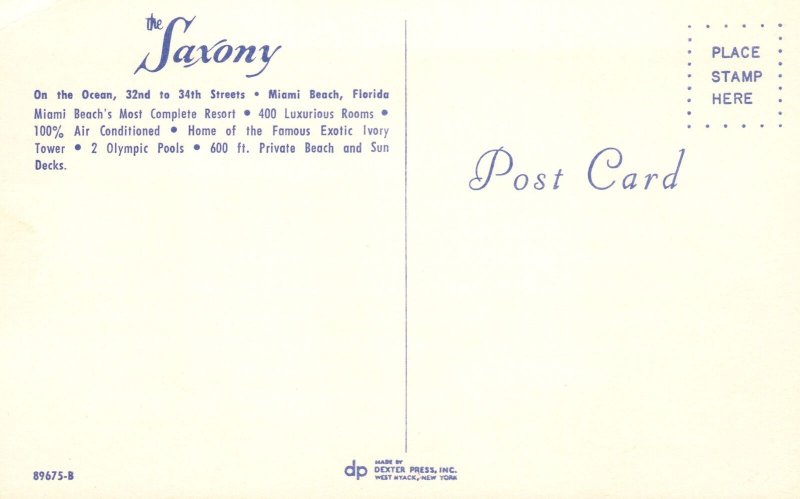The scanned image is of an old-fashioned postcard with a faded beige-white background and blue text. The back of the postcard is divided into two halves. On the right side, the word "POSTCARD" is centered in ornate lettering, with the P and C particularly elaborate. The upper right corner has a square outline labeled "Place Stamp Here" in blue text. The bottom corner features the text "Dexter Press Incorporated, West Nyack, New York" along with the company's logo marked "DP" and a code number "89675-B". 

The left side of the postcard introduces "The Saxony" in fancy writing, detailing it as "Miami Beach's most complete resort" located "On the Ocean, 32nd to 34th Street, Miami Beach, Florida." The text provides an enticing description of the hotel, boasting "400 luxurious rooms, 100% air-conditioned," as well as being "home of the famous exotic Ivory Tower." It also highlights amenities such as "two Olympic pools, a 600-foot private beach, and sun decks."